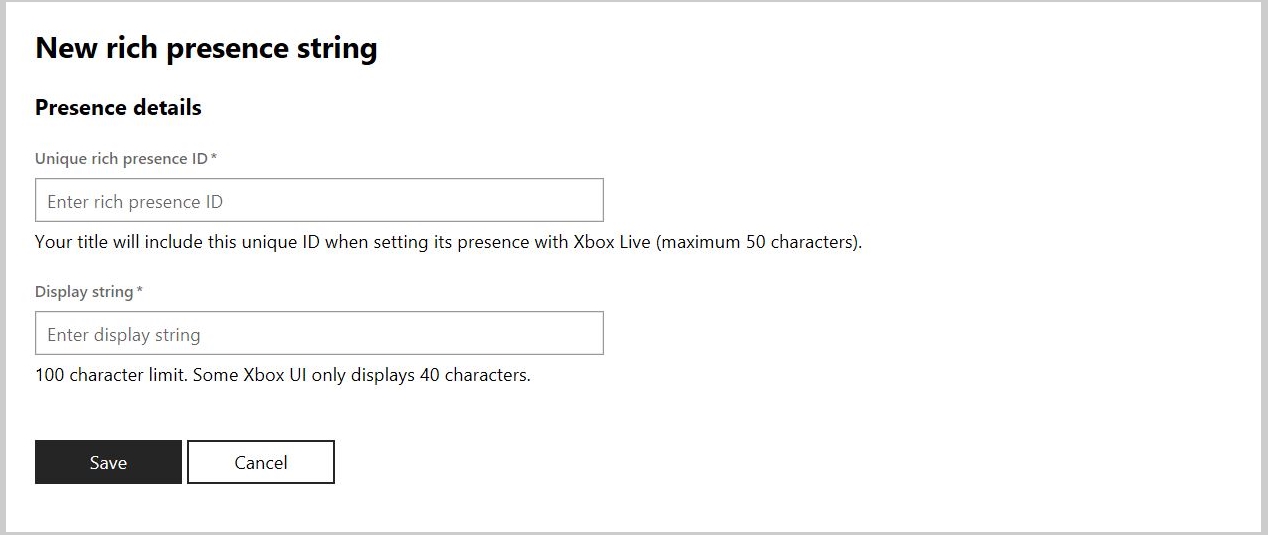The image portrays a minimalist interface design on a white background characterized by dark-colored text and devoid of any decorative elements such as images or logos. In the top left corner, there is text in black font that reads "New Rich Presence String." Below this heading, slightly smaller black text reads "Presence Details." Underneath, in a darker gray font, the phrase "Unique Rich Presence ID*" is displayed, followed by a long rectangular text box with the placeholder text "Enter Rich Presence ID" in gray. Directly below the text box, there's a note stating, "Your title will include this unique ID when setting its presence with Xbox Live. Maximum 50 characters."

Continuing further, additional gray text reads "Display String*," followed by another long rectangular text box containing the placeholder text "Enter Display String." Beneath this text box, there's a note specifying, "100 character limit. Some Xbox UI only displays 40 characters." At the bottom of the page, two interactable rectangles are present. The first rectangle has a black background with centered white text that reads "Save." The adjacent rectangle features a white background with a black border and centered black text that reads "Cancel."